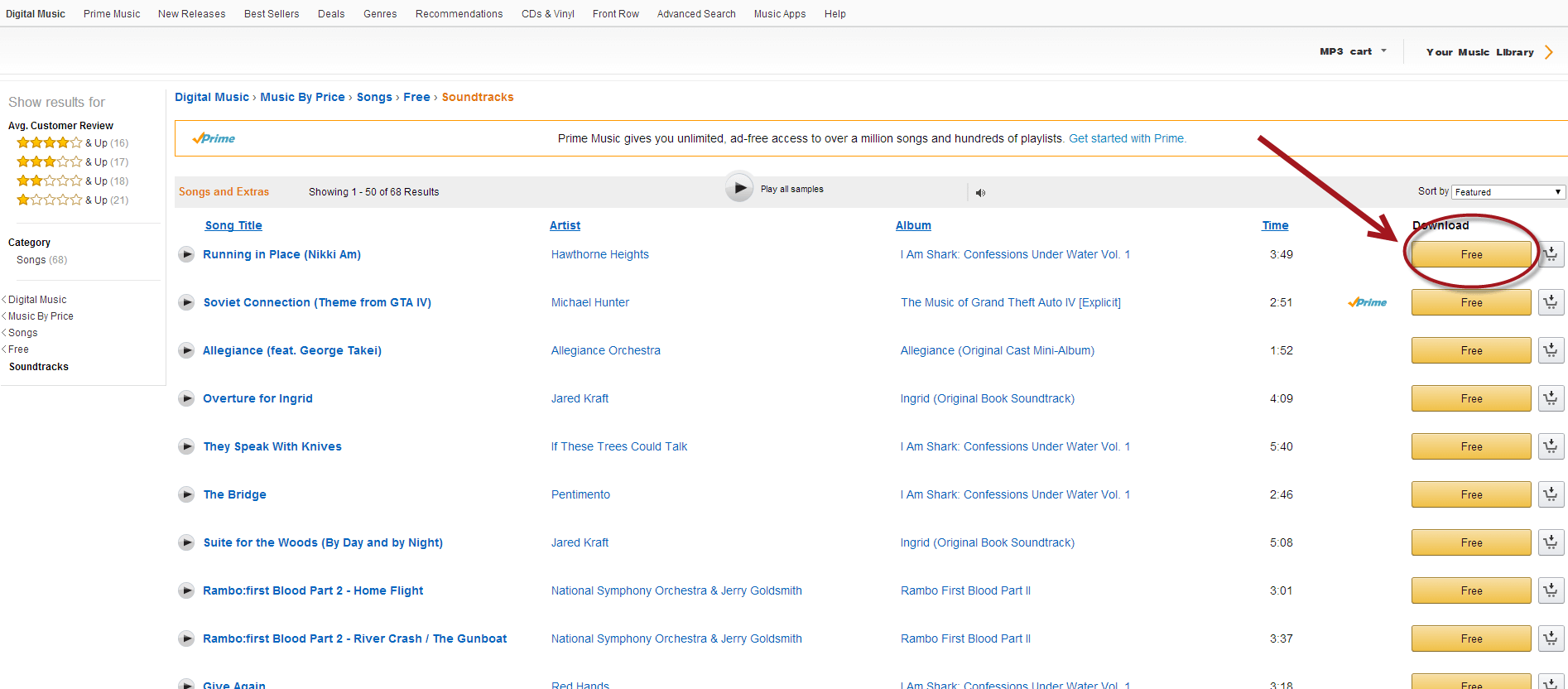This image is a landscape-oriented photo of a screenshot displaying search results on a computer or laptop screen. At the very top of the image, there is a gray-bordered header with black text reading "Digital Music." This main header is followed by subheaders that include "Free Prime Music," "New Releases," and various other recommendations that are difficult to read clearly.

Directly below this header, another gray border spans horizontally across the screen. Within this section, there is a drop-down menu labeled "Cart," and next to it, text reading "Your Music Library" in black, accompanied by a yellowish-orange right-facing arrow.

On the left side of the screenshot, there is a sidebar titled "Show Results For," which includes a category for "Average Customer Review" with different star ratings, followed by additional categories and subcategories.

At the top of the main content, the navigation pathway is shown in blue text and reads "Digital Music > Music > By Price > Songs > Free," leading to an orange-highlighted "Soundtracks" section. An orange rectangular banner with the "Prime" icon extends horizontally across the screen, indicating that these songs are available for Prime members.

Further down, there is a header labeled "Songs and Extras." Below this header, columns are organized in blue text under the headings "Song Title," "Artist," "Album," "Time," and "Download." Each "Download" item is enclosed within a yellow rectangular box that contains black text reading "Free."

Attention is drawn to the top item in the list, which is highlighted with a red circle and an arrow pointing towards it, emphasizing its importance or relevance in the search results.